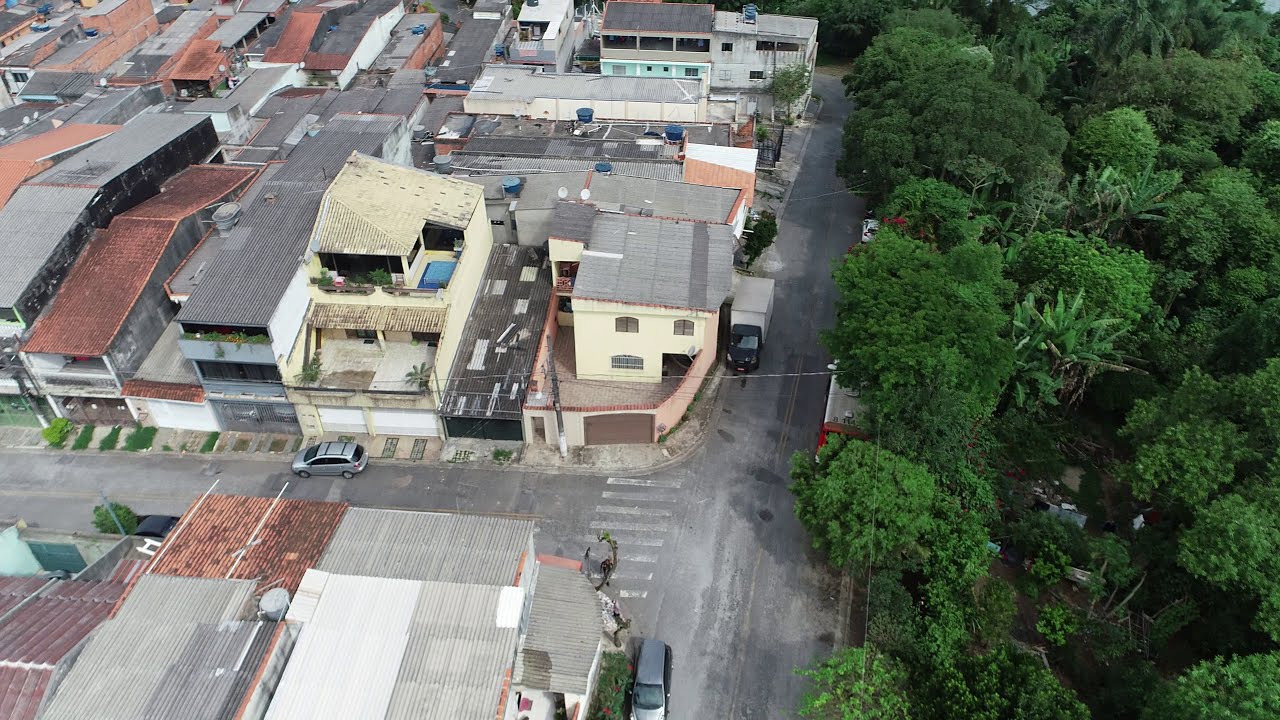The image captures an outdoor setting from an aerial perspective, resembling a bird's-eye view. On the right-hand side, a dense forest of lush, green trees occupies about a third of the frame. Some of these trees have palm leaves, adding a tropical feel to the scene. The trees cast noticeable shadows onto a worn road that edges between the forest and the residential area. This road runs vertically along the tree line, while another road cuts horizontally between the buildings.

The left side of the image reveals a residential area filled with numerous multi-story buildings, mostly ranging from two to four stories high. These structures are closely packed together and feature a mix of flat, metal roofs in gray and reddish clay colors. Some buildings boast terraces, occasionally adorned with plants, while others remain open. The roads weaving through this area appear worn, with a zebra crossing that is also faded. Several vehicles are sporadically parked along these streets. The environment looks dry, and although it is daylight, the lighting suggests an overcast or not particularly bright day, with no visible sun in the frame.